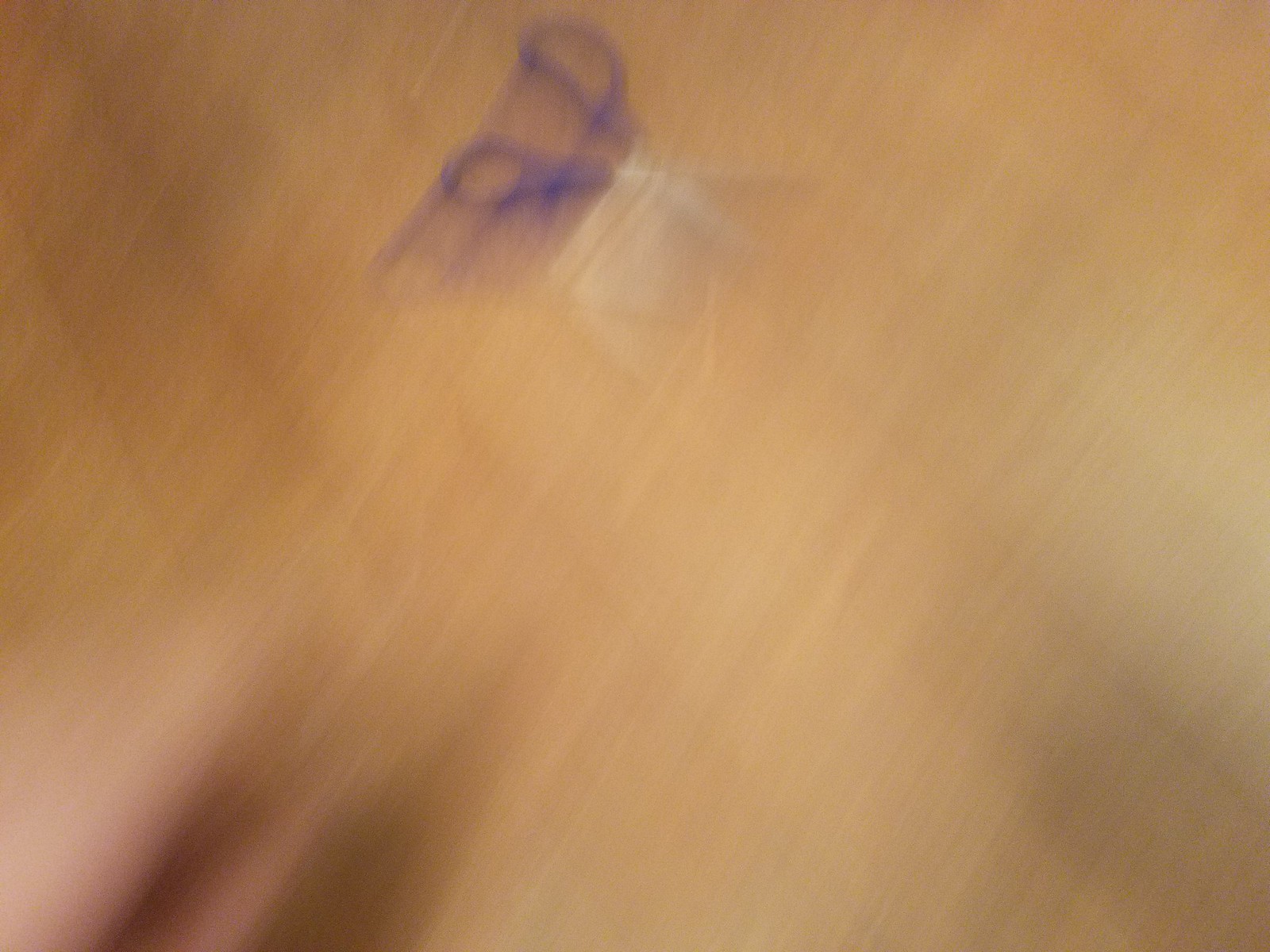This image is an extremely blurry, almost unrecognizable photo of an open pair of scissors lying on a wooden table. The scissors, which feature silver metal blades and dark blue or dark purple plastic handles, are positioned with their handles pointing towards the top edge of the image and their blades extending towards the bottom right. The background consists of a blurred, light brown wooden surface, characterized by diagonal stripes suggesting a wooden texture. At the bottom left corner, there is a blurry hint of a hand, with faint flesh tones and indistinct features. Additionally, some shadows and areas of light purple hue are visible around the left side of the image, contributing to the overall out-of-focus appearance. The extreme blurriness creates the effect of the scissors’ colors continuing towards the left side.